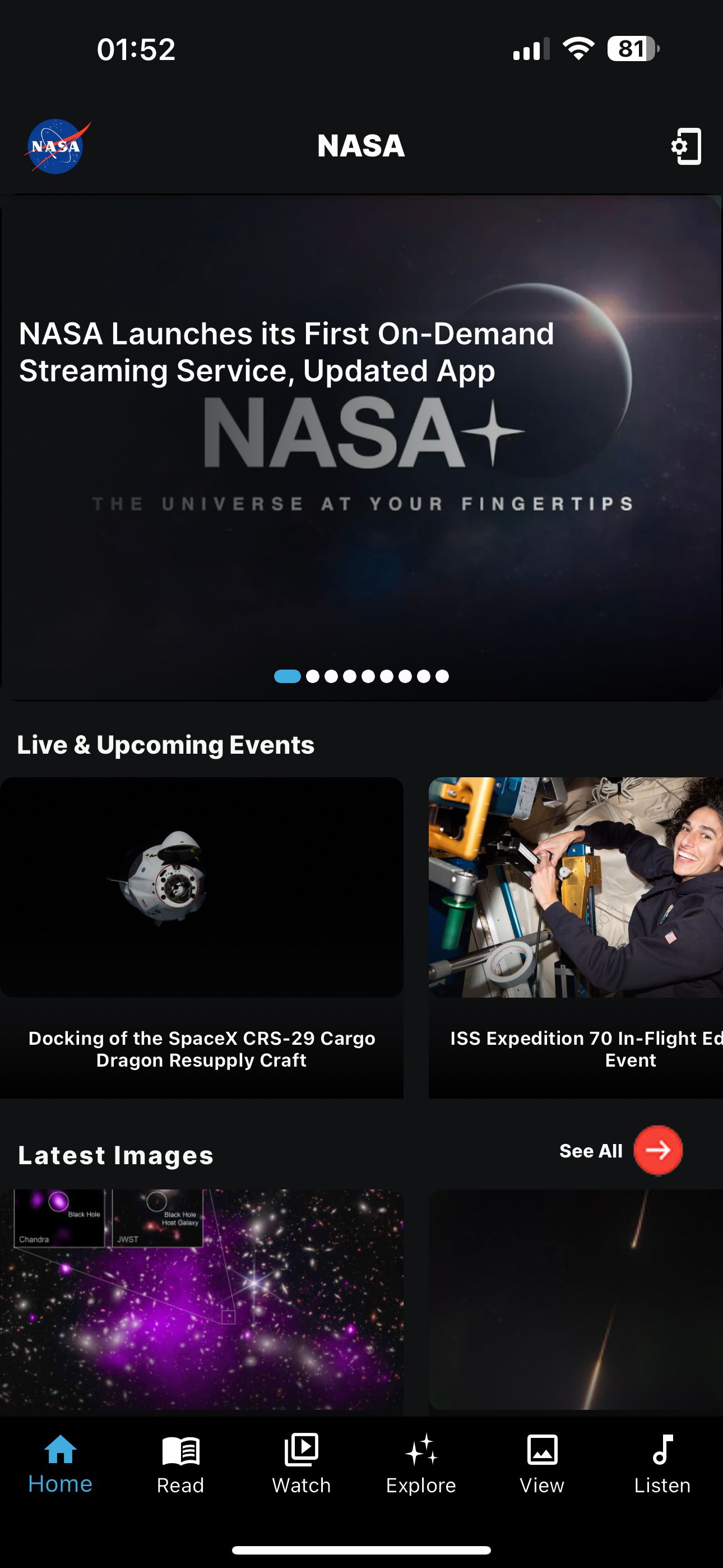Here is a cleaned-up and detailed caption for the given image:

---

This is an image of a NASA webpage featuring the "Blue World" logo with a red arrow going through it, accompanied by the NASA insignia at the top. The page announces the launch of NASA's first on-demand streaming service with the headline, "NASA Launches its First On-Demand Streaming Service." The updated app is described as "NASA Plus: The Universe at Your Fingertips." The interface includes several sections of information such as live and upcoming events. One highlighted event is the docking of the SpaceX CRS-29 Cargo Dragon resupply craft, illustrated with an image of the spacecraft. Another section features an image of an astronaut, possibly aboard the spacecraft, alongside the caption "ISS Expedition 70 In Flight" with the word "Event" beneath it. Additionally, the page showcases the latest images, featuring a stunning star-studded sky set against a purple background, with a link labeled "See All" for further exploration.

---

This caption provides a detailed and cleaned-up description of the contents and layout of the image, offering clear information for the reader.